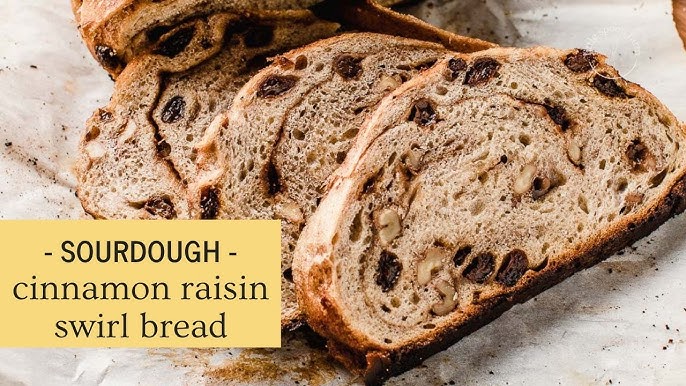This horizontal, close-up color photograph showcases three slices of sourdough cinnamon raisin swirl bread, prominently occupying the majority of the frame. The bread, with its dark brown crust, is laid flat and slightly overlapping on a white cooking paper that features scattered crumbs. The interior of each slice reveals intricate swirls of cinnamon, interspersed with visible brown raisins and white nuts. The image is so detailed that one can discern individual air bubbles and fibers within the loaf. At the bottom left corner of the photo, a pale yellow rectangle contains black text that reads "sourdough cinnamon raisin swirl bread." Behind the slices, the remainder of the loaf is just barely visible.